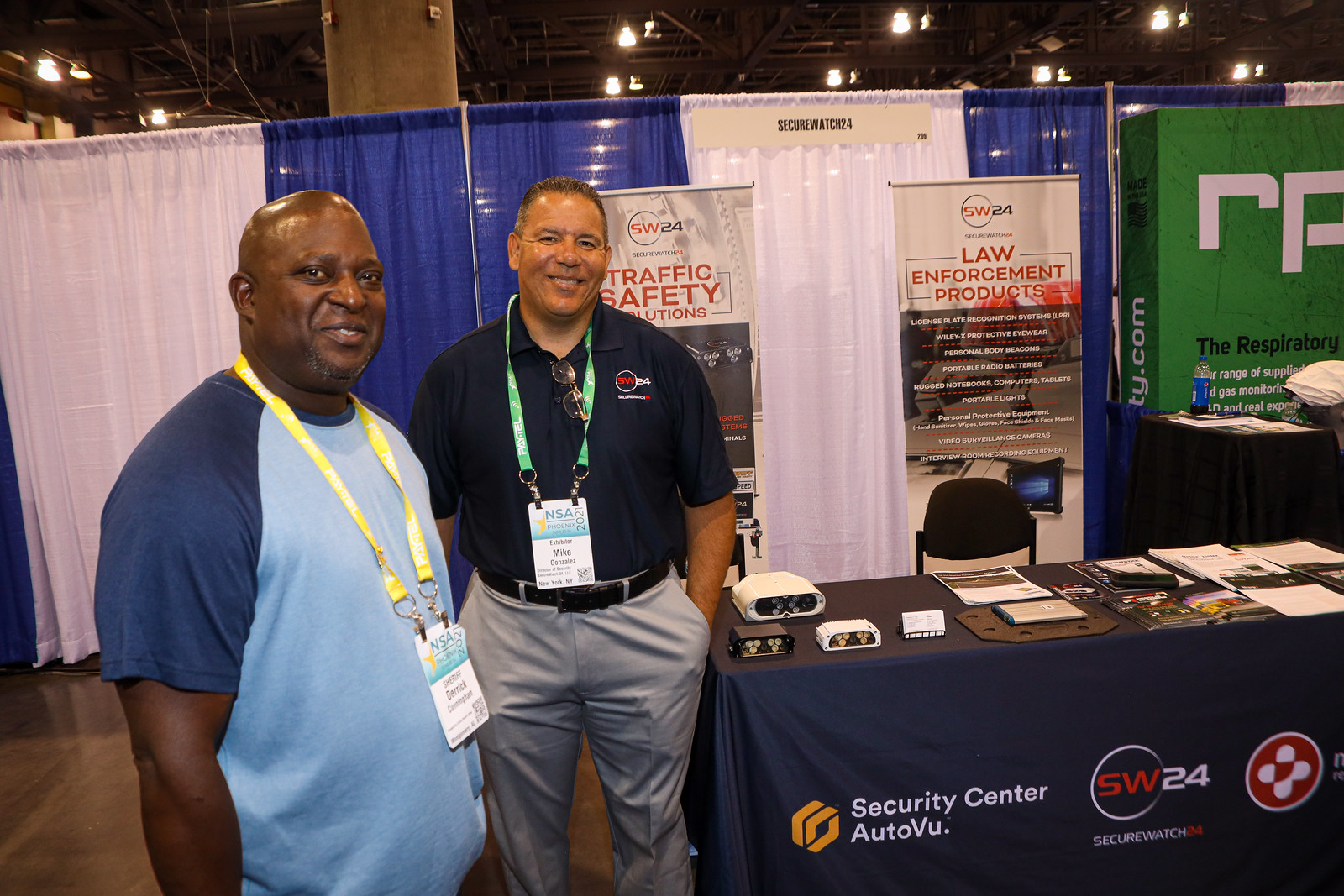In the image, two men are standing at a booth promoting law enforcement products, likely at a conference or trade show. The man on the left, an African American with a bald head, is wearing a light blue shirt with dark blue sleeves and a yellow NSA lanyard around his neck. He is smiling warmly. To his right is a Hispanic man with some graying hair, also smiling. He is dressed in a dark blue polo shirt bearing a logo and has sunglasses hanging from his shirt collar. He is wearing a green NSA lanyard, and his dark blue polo shirt is neatly tucked into white slacks, secured with a black belt. Behind them, the booth is adorned with blue and white curtain-like dividers and multiple signs indicating "SW-24 law enforcement products," "Security Center," "Auto," "Blue," "SW-24," and "Secure Watch 24." Despite some text being small and illegible, the booth's table displays various branded materials, including pamphlets and what resemble virtual reality headsets in white, black, and cream colors. A black chair is positioned behind their table, emphasizing the booth setup.